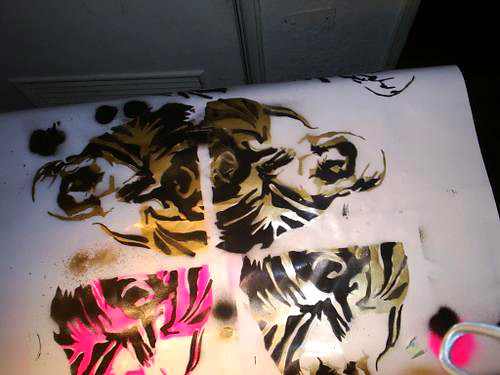A close-up image features an abstract, free-form painting on a white canvas, prominently using bold colors such as black, gold, hot pink, light brown, and orange. The artwork includes different shapes and stripes, with sections on the left side showcasing primarily orange, black, and white, while the top and bottom sections mix pink, black, and white. The right side features mainly brownish black and white hues. Among the patterns are elements resembling tiger stripes, and at the bottom right corner, a pink circle with a black dot and a loop design are noticeable. The canvas appears slightly curled or rolled at the top, giving it a dynamic look. In the background, a nearly closed door with a grated bottom and a wall with a light switch is visible, along with what seems to be lockers further accentuating the scene.